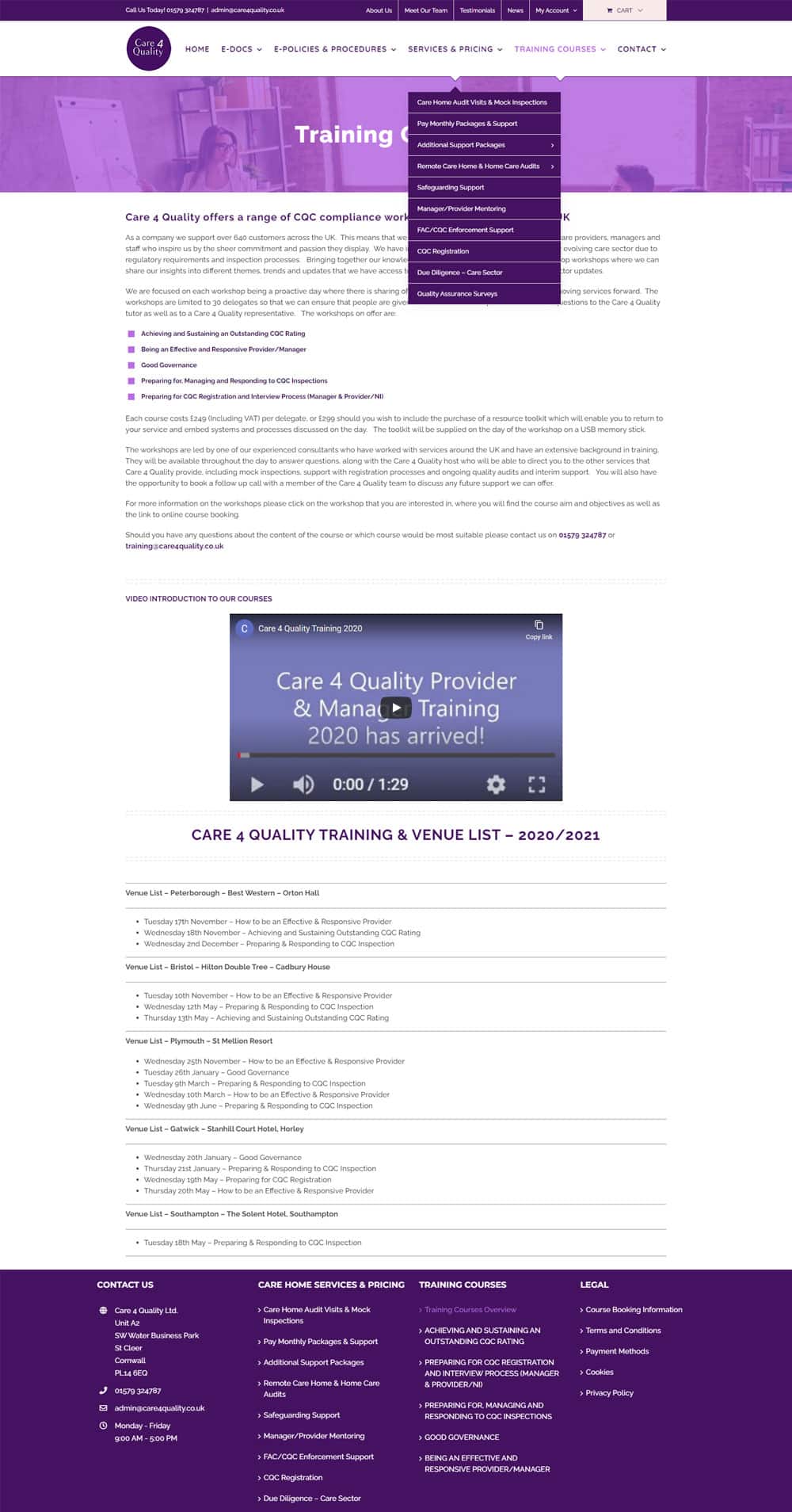The "Care for Quality" website exudes a cohesive theme of purple and white, embodying a professional and cohesive aesthetic. At the top of the page, a bold purple border hosts white text, ensuring clear visibility. Below this, the main body of the site displays a clean, white background accentuated with purple text. A visually engaging section follows with a light purple backdrop and prominent white text, featuring an image of an individual.

The content reads: "Care for Quality offers a range of COC Compliance", highlighted in purple font, followed by detailed bullet points also in purple, elaborating on the various services provided. Further down, the site presents a video section under the purple header: "Video Introduction to Our Courses". The embedded video titled "Care for Quality Provider and Manual Training 2020" stands out against its purple background with white text, inviting users to explore their offerings.

Continuing, another purple header announces: "Care for Quality Training and Venue List 2020-2021", leading to a list of approximately five venues. Towards the bottom, a purple box with white text provides information on contacting the company, care home services, pricing, training courses, and legal services, with each section offering multiple navigational options.